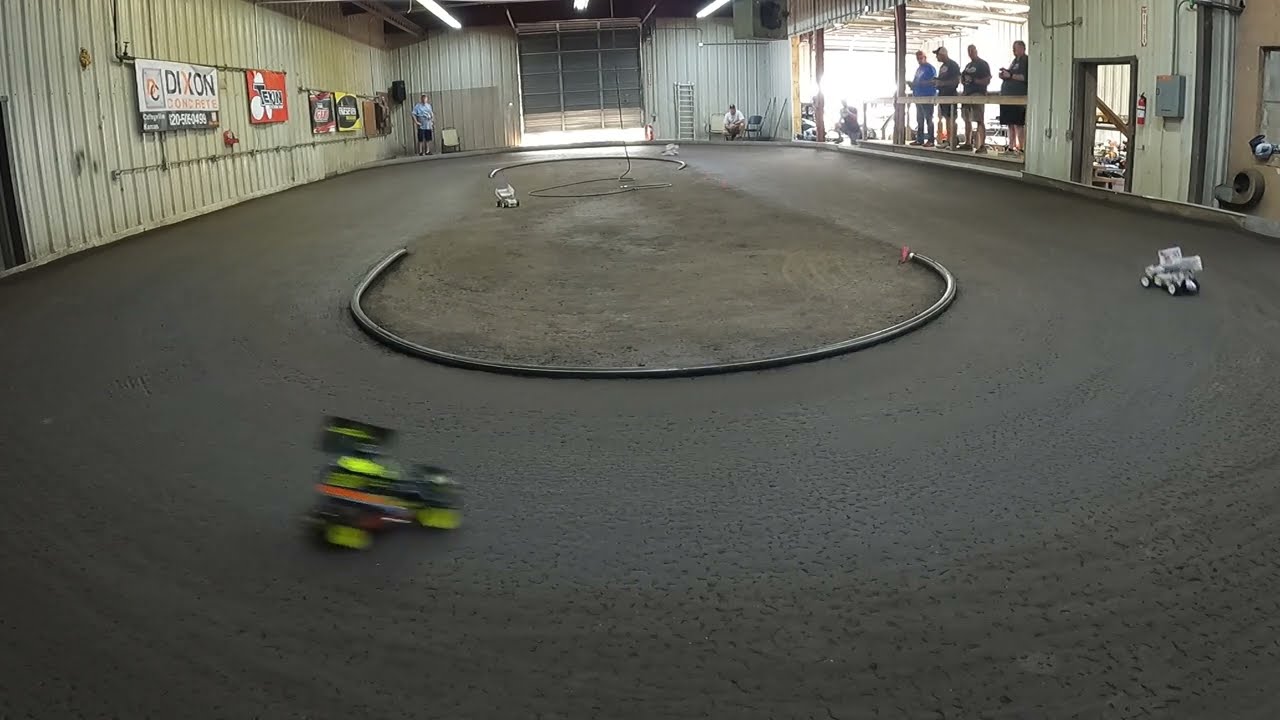This color photograph depicts an indoor remote-controlled car racetrack within a warehouse-like sporting facility. The track, made of rough, dark gray concrete with numerous small holes, features a central gravel-filled oval island where vehicles can be rested. There are two RC cars currently on the track: a white one leading on the right side and another white one in the upper right. Additionally, a black, yellow, and orange RC car appears blurred in motion in the lower left corner. The room's right-hand side has a beige corrugated wall adorned with illegible posters and a large window with a balcony. Four men stand there, two holding remote controls and watching the race. In the background, two more individuals are seen observing from the left and right sides of the room. The scene is captured in landscape orientation, emphasizing a photographic realism style.